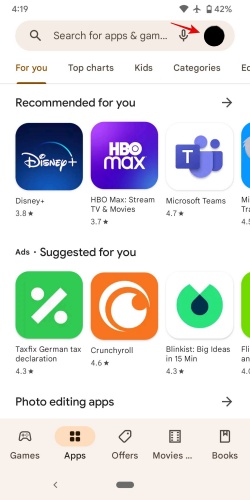Here is a cleaned-up and detailed descriptive caption for the image:

---

The image shows a phone screen with the battery at 42% and the device set to airplane mode, indicating a strong connection. The time on the phone is 4:19. At the top of the screen, a search bar labeled "search for apps and games" is adorned with a red downward-pointing arrow leading to a black circle, which overlaps with a microphone icon. 

Below the search bar, the navigation tabs read: "For You," "Top Charts," "Kids," and "Categories," with another partially visible tab labeled "EC." The section labeled "Recommended For You" lists various app suggestions, including "Disney," "HBO," "Microsoft Teams," and "Tax Fix German Tax Declaration." 

Additionally, there is an app with a partially visible blue icon, followed by "Crunchy Roll," which is represented in orange with white swirls, and "Blinkist: Big Ideas in 15 Minutes," displayed in green and black. Another app, colored green, is partially cut off and not identifiable.

At the bottom of the screen, various categories are listed: "Photo Editing Apps," "Games," "Apps," "Offers," "Movies," and "Books," with the "Apps" category currently highlighted.

---

This caption provides a clear and detailed description of the phone screen, its status indicators, and the visible content.